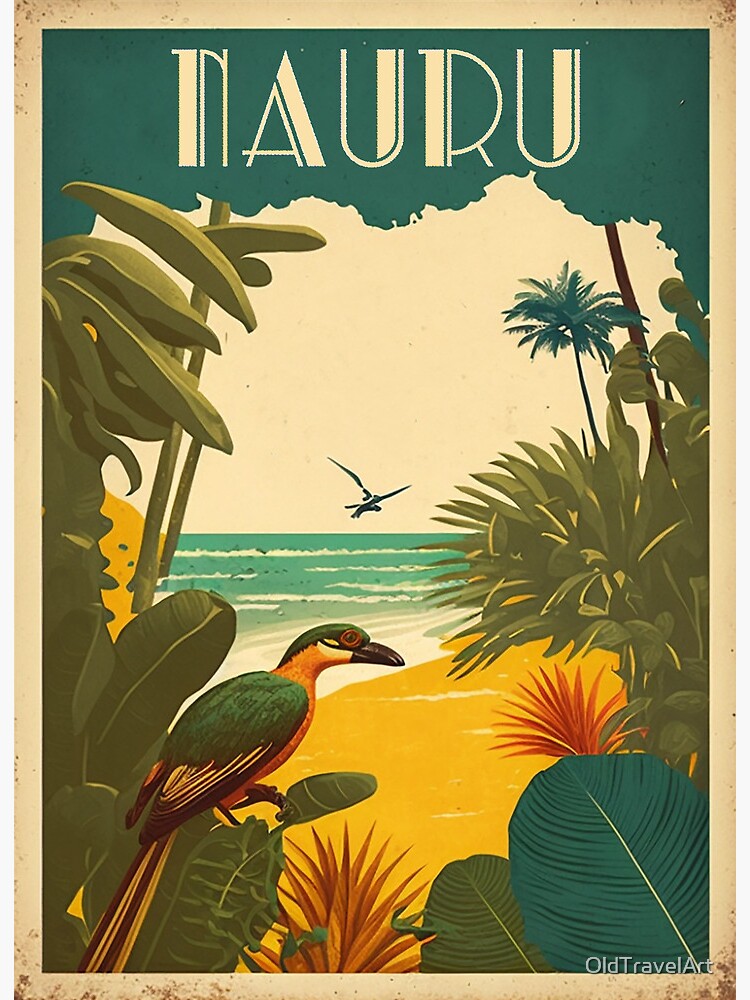This vibrant, full-color travel postcard art, titled "Nauru" in an elegant Art Deco font at the top, depicts a picturesque tropical beach scene. The postcard's design, embellished with a decorative border featuring shades of green, orange, yellow, and ivory, evokes a vintage charm, enhanced by a white border with subtle brown splatters that simulate aging. 

In the scene, the central focus is a vividly colored tropical bird perched on lush green foliage. This bird, characterized by its striking green wings, orange belly, orange neck, and long black-and-yellow tail, has a short black beak and a green head adorned with a yellow spot. 

The beach setting, seen in the background, showcases pristine yellow sand, a blue ocean with gentle white-capped waves, and a seagull soaring gracefully in the sky. Both sides of the beach are adorned with various tropical plants, including palm trees, green ferns, large elephant-ear leaves, and orange flowers, creating a lush, inviting atmosphere. The entire scene captures the serene and exotic allure of Nauru.